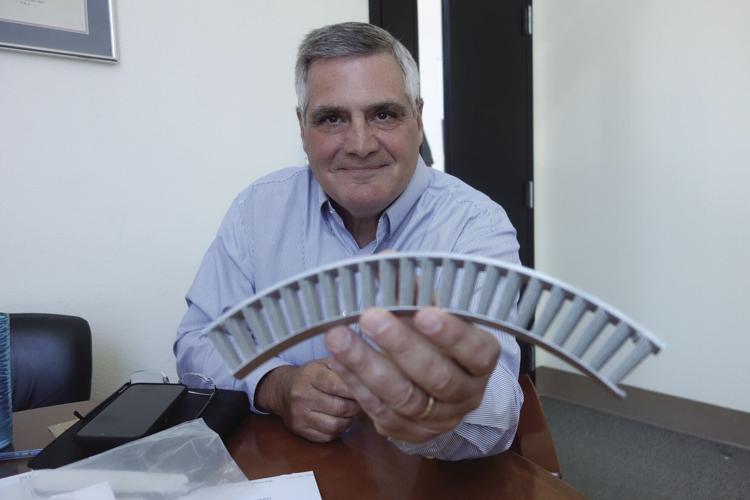In the photograph, a man is seated at a brown, office-like table. He is dressed in a long-sleeved, light blue button-up shirt, and his salt-and-pepper hair is neatly combed, darker gray on the top and lighter gray on the sides. The man, facing the camera and smiling, holds a green, semi-circular object that resembles a curved piece of toy train track or a bent arched ladder. His hands rest on the table, where a pair of glasses, his cell phone, and possibly an iPad with a black leather case are also placed. The wall behind him is painted white, with a black partially open door in the center and a picture hanging on the upper left. Additionally, a black leather chair back is visible to the left, alongside some crumpled tissue paper and what appears to be a corner of printer paper. The man wears a gold band on his wedding finger.